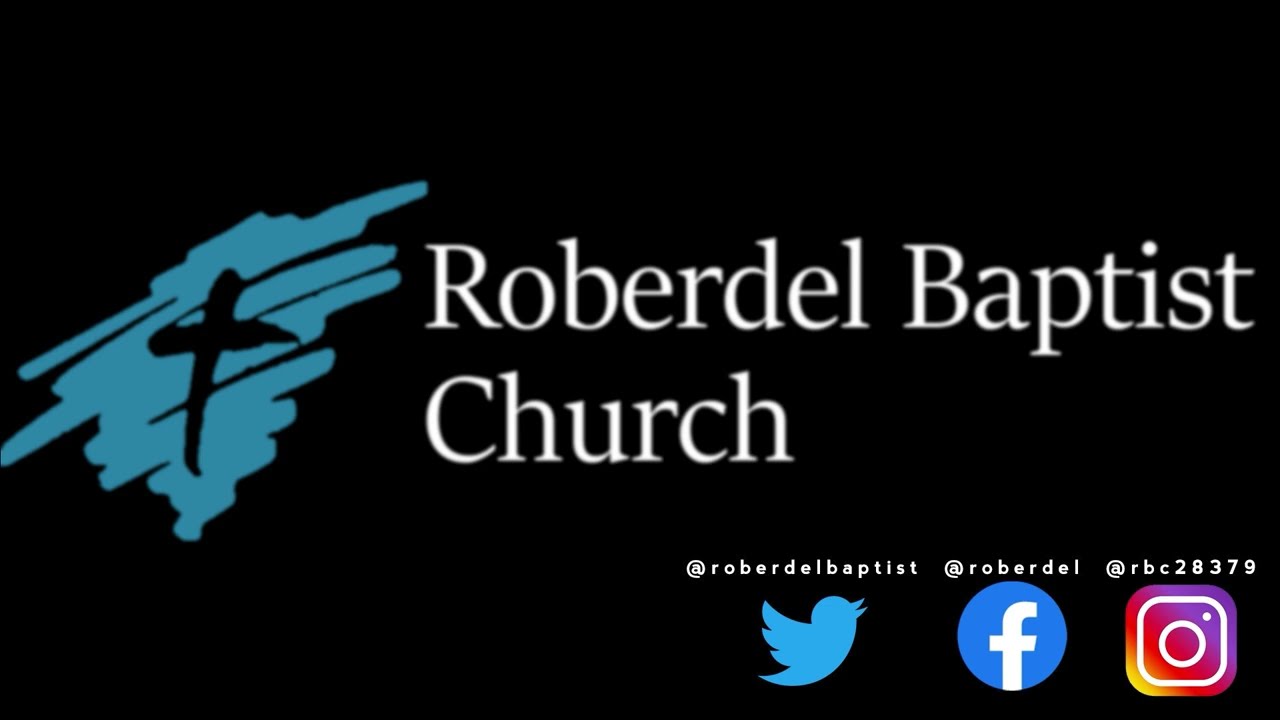The image is a professionally designed banner for the Roberdel Baptist Church, ideal for a website or social media platform. With a pure black background, this image features prominent white lettering that spells out "Roberdel Baptist Church" (R-O-B-E-R-D-E-L) in a tall, 16 to 18-point font. Positioned to the left of the text is the church's logo, which consists of blue, handwritten-like squiggly lines serving as a background for a central black cross. In the bottom right-hand corner of the image, there are enlarged social media icons linking to the church's established accounts. From left to right, these icons include Twitter (@RoberdelBaptist), Facebook (@Roberdel), and Instagram (@RBC28379). The overall dimensions of the image are approximately 8 inches across by 6 inches tall, and it contains no borders or additional objects, ensuring a clean and professional appearance.